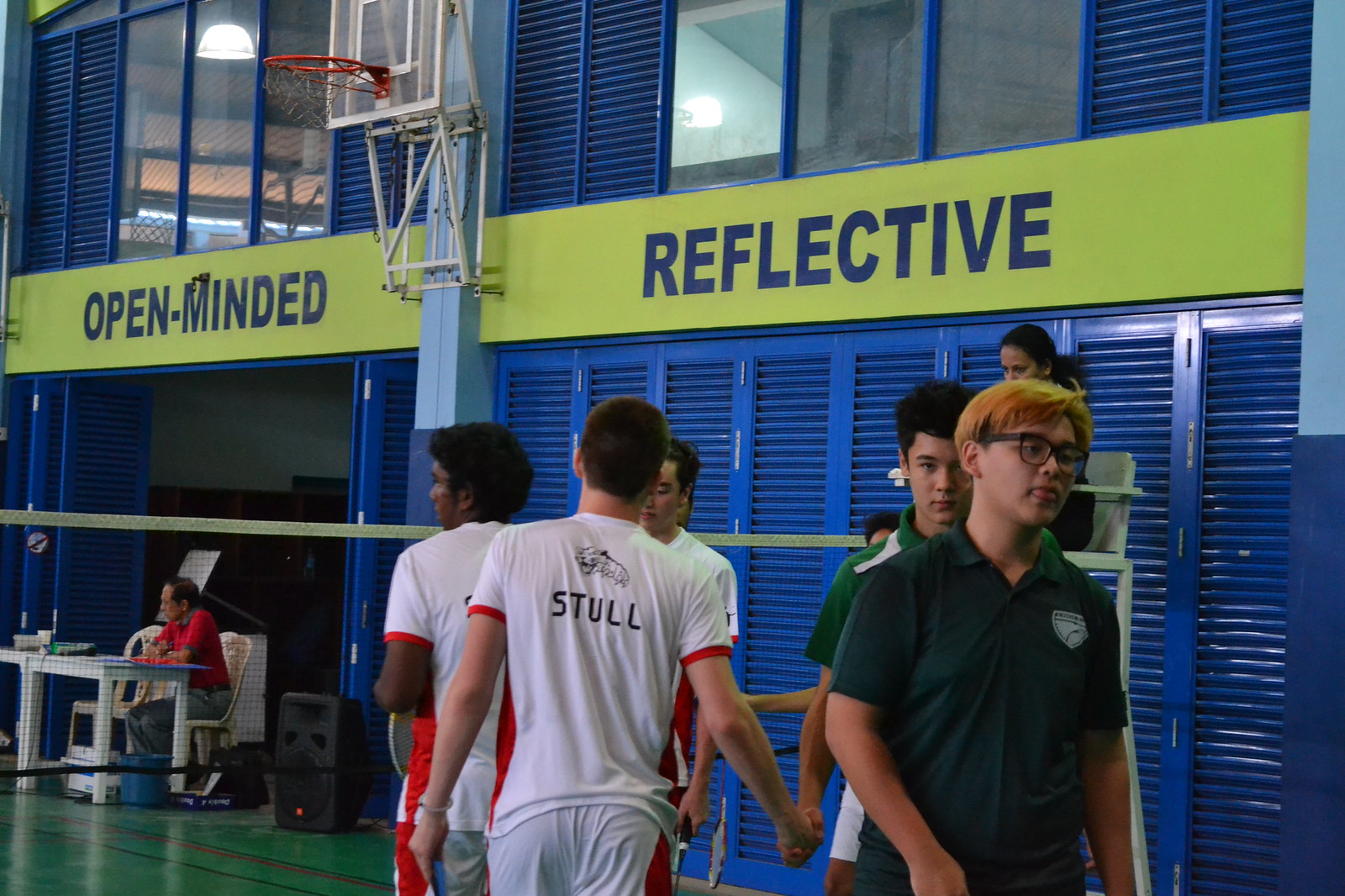The rectangular photograph captures the interior of a school gymnasium, featuring two levels of walls lined with blue shutters that can open and close. The gym's focal point is highlighted by a lime-green banner with blue text reading "open-minded and reflective," suspended in the middle of the wall. Below this sign, a basketball hoop, currently pulled up and unusable, is also visible.

In the foreground, a volleyball net stretches from right to left, dividing the space. On the court, several players, likely teenage boys, huddle together. One team wears white jerseys with red trim, while some individuals in green polo-like shirts stand nearby. A referee is seated in a high chair, overseeing the game. Additionally, on the left side of the image, a man in a red shirt sits at a white desk, presumably scorekeeping, with some exercise equipment visible in the background on the second floor. The entire scene captures a moment of preparation or discussion, rather than active play.